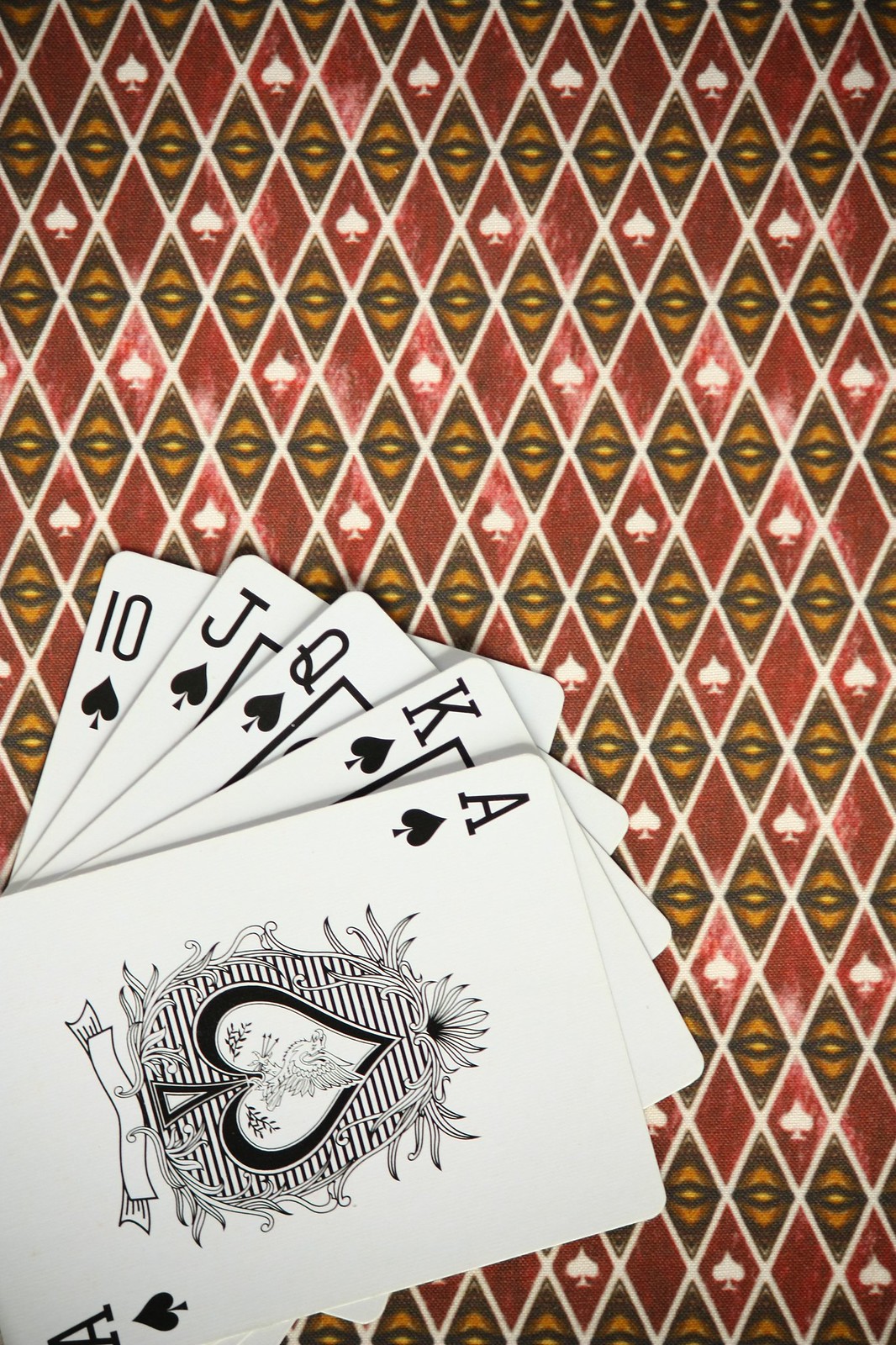In the close-up image, a beautifully fanned-out hand of poker cards is displayed on a richly patterned table. The table surface features a repeating diamond pattern, with each diamond outlined in white. Some diamonds are filled with a dusty red color, while others house a white spade symbol on a red background. Additionally, rows of diamonds contain an intricate gold design resembling an eye, complete with an upper and lower lid, a pupil, and an iris filled in black.

The cards, which are white and face up, reveal a stunning array of spades. At the forefront is the ace of spades, showcasing a large, elaborate spade design in black and white. The spade itself has a thick black border with an inner white spade, accompanied by a horizontally pinstriped black and white motif resembling a stylized pineapple, adorned with leafy embellishments.

Beneath the ace of spades are the king, queen, jack, and ten of spades, each card neatly aligned and forming an elegant fan spread across the table. The ensemble creates a striking visual against the detailed backdrop, highlighting the artistry of both the cards and the patterned surface they rest on.